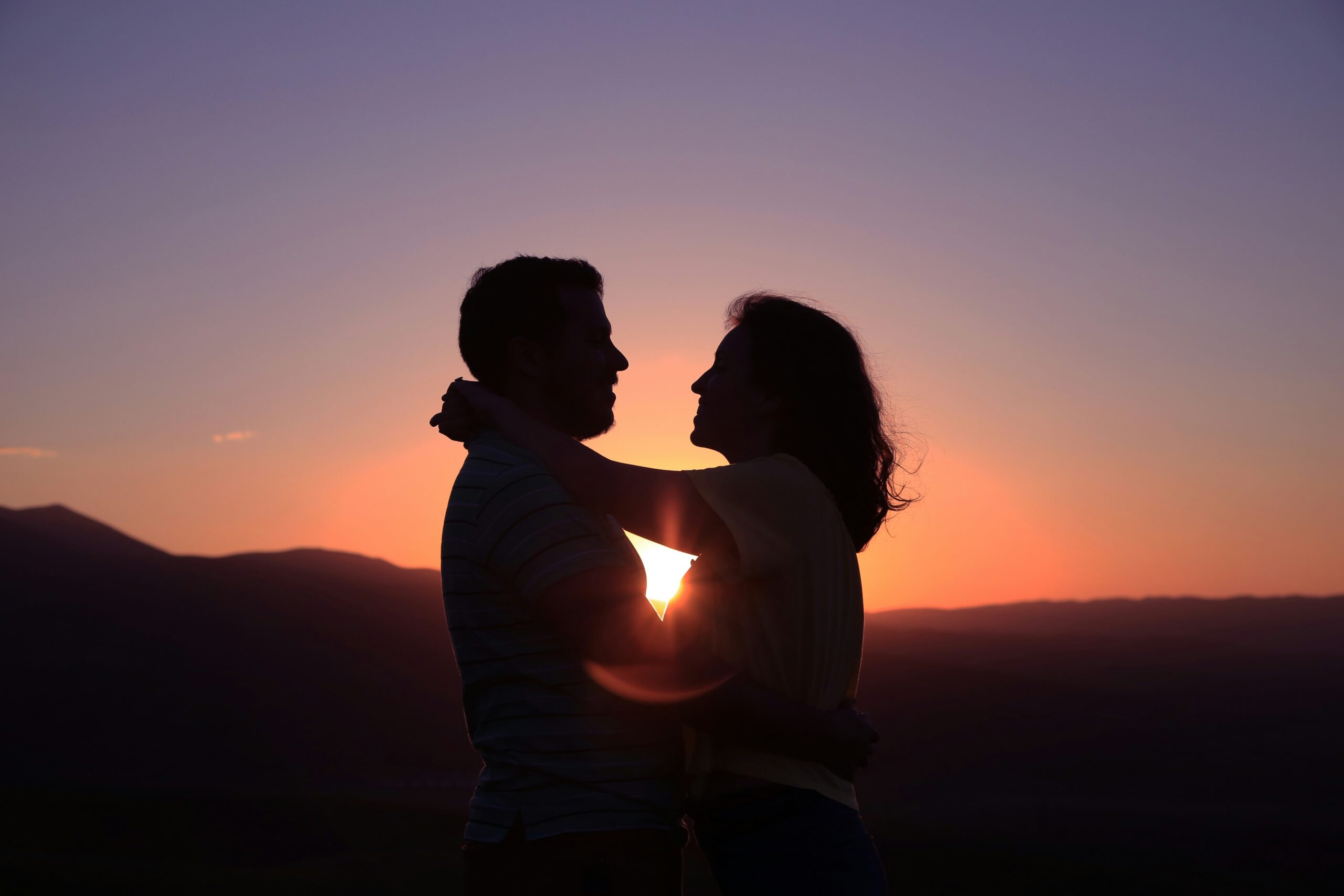In this captivating image, a couple is seen embracing in front of a vibrant sunset. The woman, with her dark, shoulder-length hair, has her arms gently draped around the man's neck, while he, with his short hair, holds her waist. Both are gazing directly into each other's eyes, their silhouettes partially blocking the setting sun that peeks through the space between their chests. The man is wearing a striped blue top, and the woman is clad in a white top. The background showcases a breathtaking sky that transitions from a reddish hue near the horizon, blending into an orange and peach tint, and then into a gradient of purple and blue as it ascends. The landscape below features a hazy outline of mountains and rolling hills, adding depth to the serene outdoor scene. The overall ambiance of the photo is both romantic and picturesque, capturing the timeless beauty of a sunset shared between two lovers.